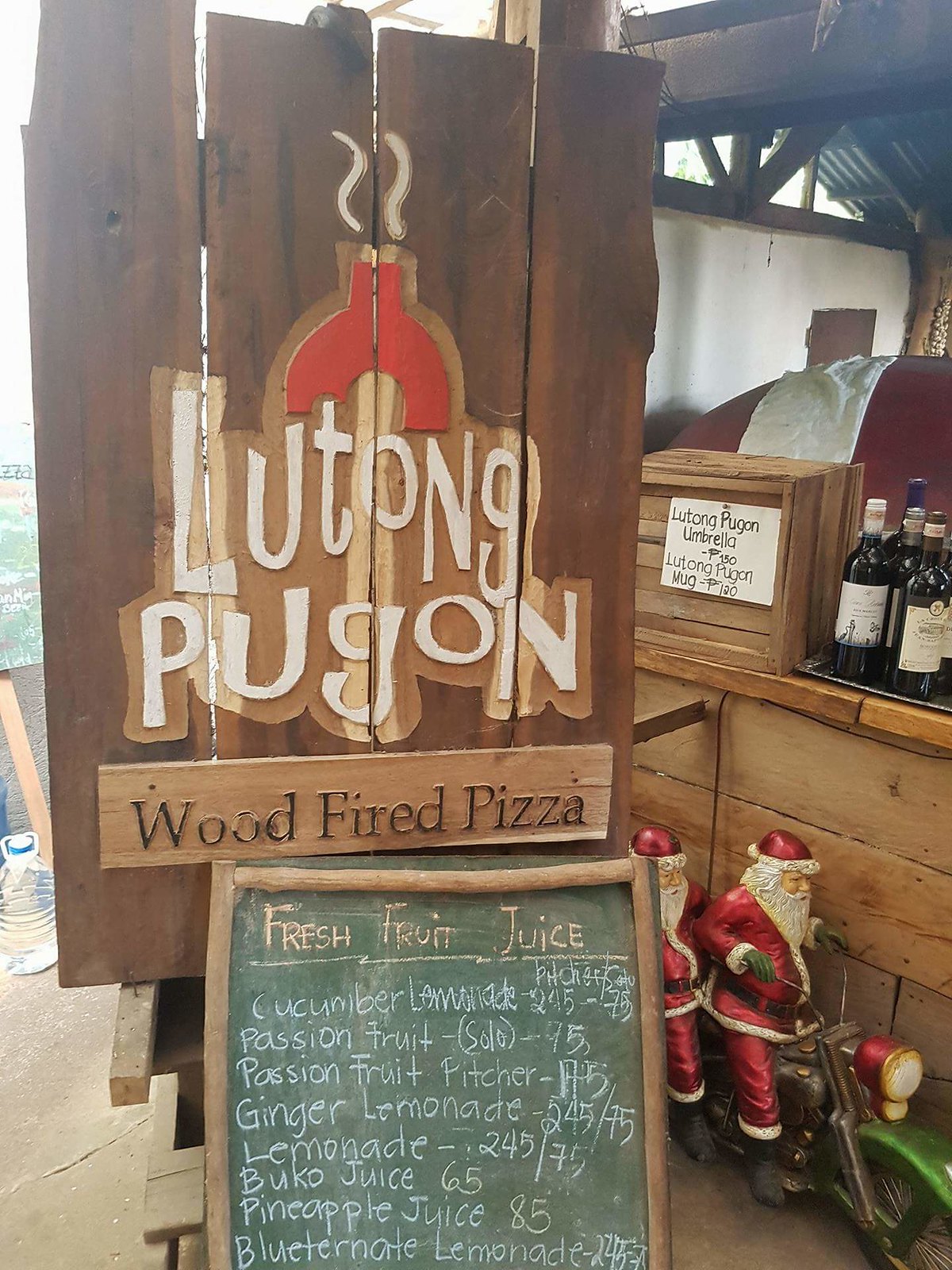This photograph captures a wooden counter likely at an outdoor restaurant or food stall. Prominently displayed on the left are four vertical wooden planks forming a sign, intricately carved with an image of a wood stove and the inscription “Lutong Pugon” in white letters, highlighting the place's specialty in wood-fired pizza. Below this, a horizontal wooden board also engraved in black reads “Wood Fired Pizza.” Beneath these signs, a green chalkboard framed in wood lists various fresh fruit juices in colorful chalk, including cucumber lemonade, passion fruit, passion fruit pitcher, ginger lemonade, lemonade, fruco juice, pineapple juice, and lutonate lemonade, with pricing detailed on the right.

Adding a whimsical touch, the counter features a statue of two Santa Clauses riding a tandem motorcycle, placed in the lower right corner. Behind them is a wooden countertop adorned with a tray of glass bottles, possibly containing beer. To the left, a small white sign promotes Lutong Pugon merchandise, listing a Lutong Pugon umbrella for $1.50 and a mug for $1.20. The setting seems open-air, as evidenced by a visible white wall with crossbeams supporting a slanted roof, providing a rustic yet inviting atmosphere for customers.